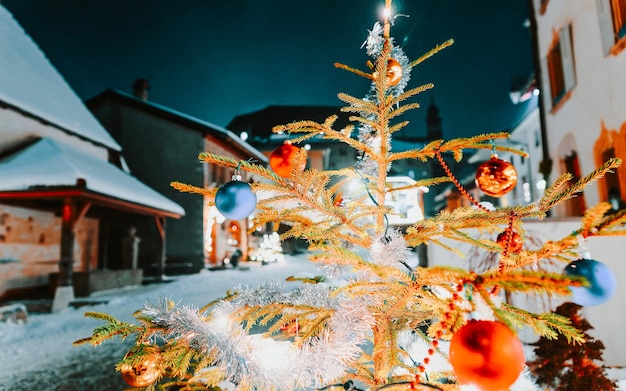In this nighttime outdoor photograph, a sparsely adorned, artificial Christmas tree stands prominently in a snow-covered village square. The scene exudes a serene, wintry atmosphere with a backdrop of slightly blurred European-style buildings. Among them, a white building with orange-outlined windows contrasts sharply with a stone building on the left, both capped with snow-laden roofs. Even further back, a taller structure with a black spire emerges.

The main focus, however, is the Christmas tree itself. Positioned centrally, its predominantly bare branches are light brown and flecked with a scanty assortment of pine needles, more concentrated towards the bottom. Wrapped around the tree are shimmering silver tinsel and strands of bright lights that illuminate the night. The decorations include an array of colorful round ornaments, primarily red and blue, in both matte and glossy finishes. Specific placements can be discerned - red baubles glisten at various lower points, while blue ones punctuate the sparse foliage. A bright light crowns the treetop, cascading more light downward.

The photograph captures the warm, festive glow of the tree against the cool, dimly lit ambient of the snow-covered town, where the dark blue sky is void of stars, slightly obscured by light pollution reflecting off the buildings.